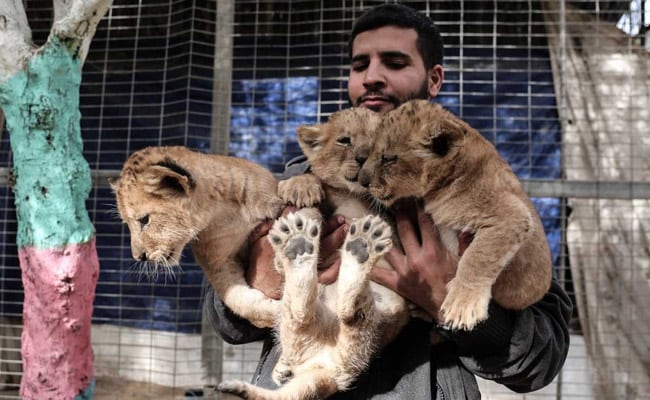The photograph depicts a seemingly Middle Eastern man in his late 20s or early 30s, dressed in a dark gray or black jacket, cradling three adorable lion cubs in his arms. The man has closely cropped black hair, a slim mustache, and a full beard, and appears to be relaxed yet focused on holding the squirming cubs. The cubs, each approximately one to two months old, have tawny, light tan fur with rounded, fuzzy ears and black pads on their paws, accented by small brown claws. The cub on the left, held in the man's right arm, leans over slightly, looking to the left. The central cub has its back pressed against the man’s chest, with its tiny forepaws looped over his hand, exposing its adorable hind feet and tail. The cub in the man’s left arm nuzzles the central cub affectionately. Behind them, there is a wired, wood-framed enclosure indicative of a zoo or refuge, and to the left of the image is a tree with a distinctly painted trunk—pink on the bottom and teal blue on the top—adding a splash of color to the scene.